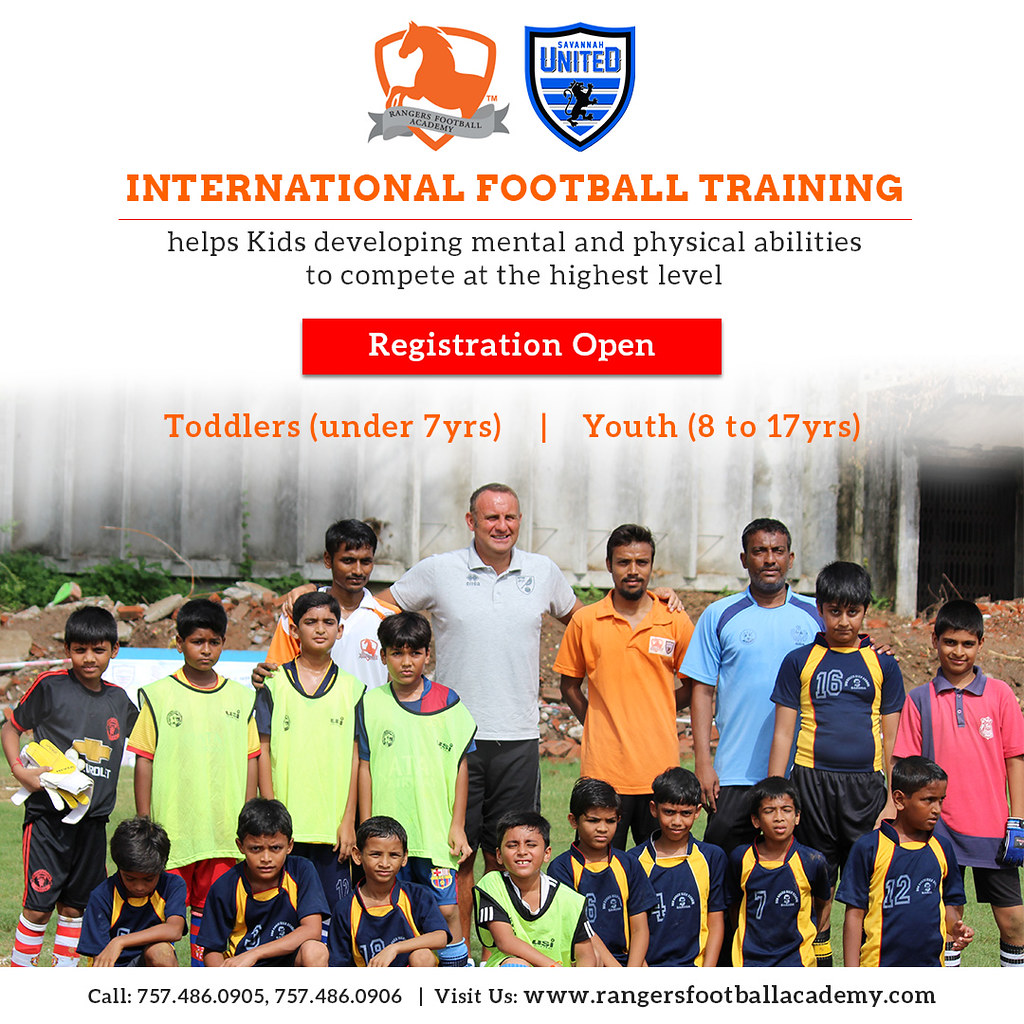The image is an advertisement for an international youth football academy. At the top, there are two prominent logos: the logo on the left features a horse jumping through a crest with the text "Rangers Football Academy," while the logo on the right displays a blue and black shield with the words "Savannah United" and a crowned lion beneath. Below these logos, the heading "International Football Training" is displayed in bold orange lettering, followed by the subheading, "Helps Kids Develop Mental and Physical Abilities to Compete at the Highest Level" in black text.

A large red rectangle beneath the text announces, "Registration Open" in white letters. Below this, the age groups "Toddlers Under 7 Years" and "Youth 8 to 17 Years" are listed in orange.

The central part of the image features a color photograph of a group of young football players, ranging in age from approximately 7 to 10 years old, wearing various shades of blue, yellow, green, and red uniforms. The back row includes four adults, likely the coaches or instructors, dressed in differing colors including orange, blue, white, and yellow. 

At the very bottom of the image, there are contact details with a phone number and the website "www.rangersfootballacademy.com."